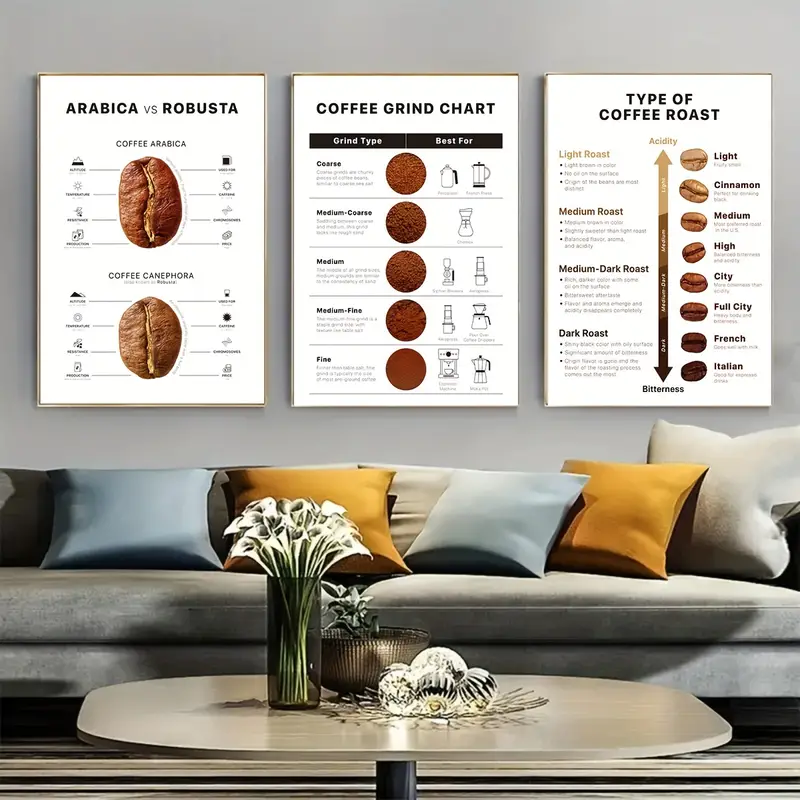The photograph captures a meticulous living room scene dominated by a central gray elongated couch adorned with blue and orange-yellow pillows. Positioned in front of the couch is a light brown coffee table that holds a gray vase of calla lilies, a bowl, and some additional ornamentation. The backdrop behind the couch is a gray wall featuring three distinct prints, each showcasing detailed aspects of the coffee-making process. From left to right, the first print discusses the differences between Arabica and Robusta coffee beans, complete with detailed labeling. The central print is a Coffee Grind Chart, illustrating various grind sizes with descriptors like coarse and medium. The rightmost print is a Type of Coffee Roast chart, depicting coffee beans from light to dark roast, with labels such as light, cinnamon, medium, and high. The overall color palette is predominantly gray, complementing the thematic coffee prints and lending a sophisticated aesthetic to the room.